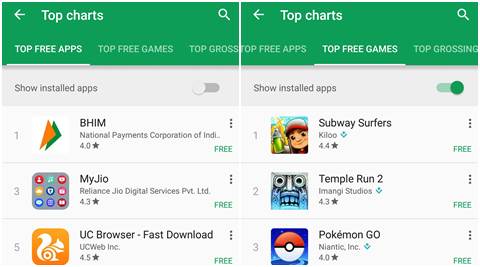This image is a screenshot from the Google Play Store, showcasing the top charts for both top free apps and top free games. 

On the left side of the image, under the "Top Free Apps" category:
1. **BHIM** - Developed by the National Payments Corporation of India. Rating not displayed. Status: Free.
2. **MyJio** - Developed by Reliance Jio Digital Services. Rating: 4.3 stars. Status: Free.
3. **UC Browser - Fast Download** - Developed by UCWeb Inc. Rating: 4.5 stars. Status: Free.

On the right side of the image, under the "Top Free Games" category:
1. **Subway Surfers** - Developed by Kiloo. Rating: 4.4 stars. Status: Free.
2. **Temple Run** - Developed by Imangi Studios. Rating: 4.3 stars. Status: Free.
3. **Pokémon GO** - Developed by Niantic, Inc. Rating: 4.0 stars. Status: Free.

Both sections are topped with a green header that includes the title "Top Charts" and a search icon. Tabs for different categories such as "Top Free Apps," "Top Free Games," "Top Grossing Apps," and "Top Grossing Games" are visible. There is also an option to filter the display to show installed apps using a toggle switch.

The layout prominently highlights the ranking, ratings, and free status of the top apps and games available for download. This screenshot appears to be from around 2015-2016.